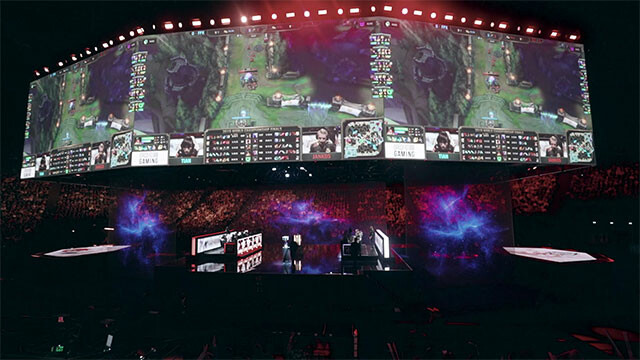The image seems to depict an indoor event, likely taking place at night, possibly a concert or a competitive gaming event held in a large auditorium or amphitheater. The dark background suggests it's either late evening or the lighting is deliberately dimmed for the event. Prominent in the top half of the photograph are three large digital screens; the center screen is flanked by two smaller ones tilted slightly backward to be more visible to the audience. The screens display players and their stats, likely indicating an ongoing arcade video game competition between a boy and a girl.

The audience is vast, with seats filled around the large venue, extending towards the back of the room. On the brightly lit stage, which is framed by the screens, several people can be seen, including the two competitors and possibly some judges sitting to their left. There are structures that look like additional stages on either side of the main stage, although they appear to be empty. Equipment such as keyboards or amplifiers are faintly discernible, adding to the technical setup for both the audience's viewing and the players' performance. The photograph captures the intensity and excitement of the event, even though the details are slightly obscured by the darkness and distance from which the photo was taken.